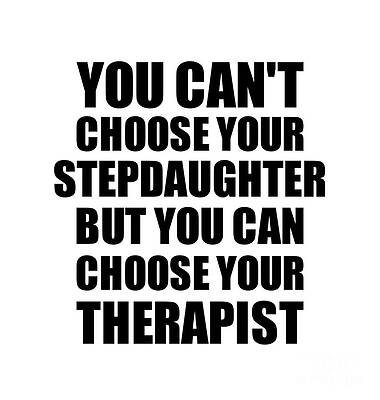The image features a simple, digitally created design with black, bulky text on a plain white background. The text is structured line by line as follows: "you can't" on the first line, "choose your" on the second line, "stepdaughter" on the third line, "but you can" on the fourth line, "choose your" on the fifth line, and "therapist" on the final line. The entire design is presented in a small square format, resembling something that might be used for a meme or a t-shirt. The message conveys a somewhat controversial and potentially offensive sentiment about the relationship between stepdaughters and therapists.